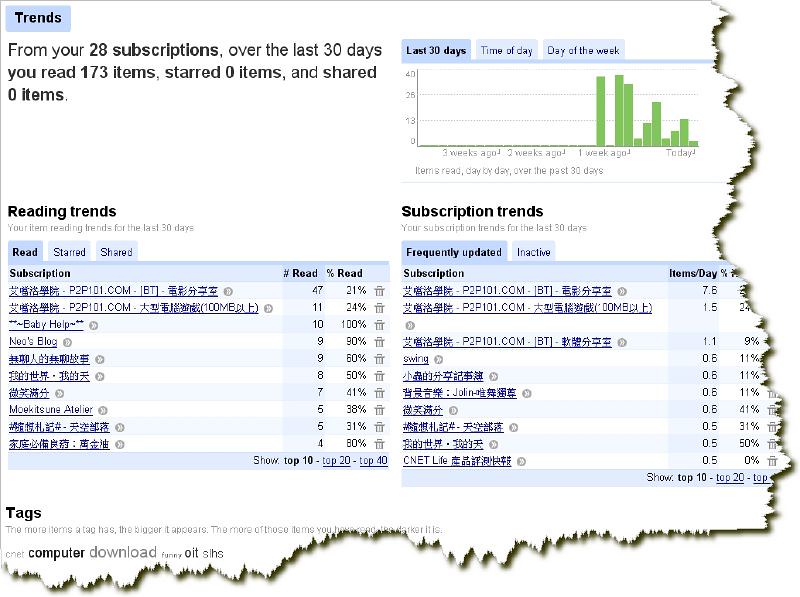This image is a detailed screenshot taken from a computer, featuring informational data about reading and subscription trends. The text is primarily in a foreign language, but key sections are in English. At the top left, it states: "Trends. From your 28 subscriptions over the last 30 days, you've read 173 items, starred zero items, and shared zero items." The central part of the image showcases various charts, including a timing chart outlining reading activity over the past 30 days. The chart visually dominates the screenshot, presenting trends and subscription data in a layout filled with white, black, light blue, green, and gray colors. No people are present in the image, and it has jagged edges, indicative of a screenshot rather than a smooth photograph. Overall, this picture represents a digital summary of reading statistics and subscription trends captured from a website.